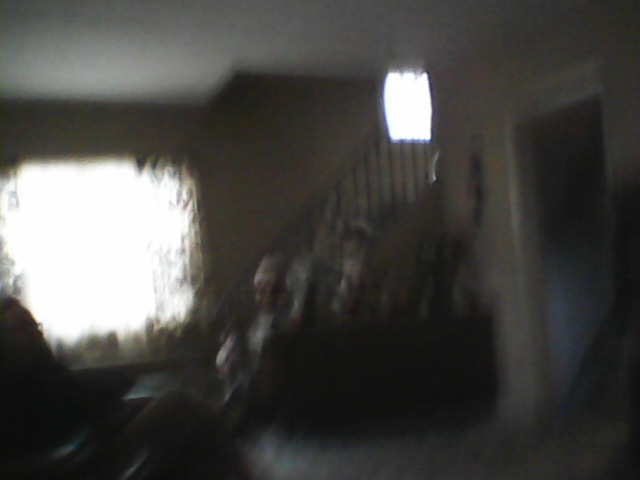This photograph, although blurry, captures a cozy interior of a home. The top portion of the image starts with a white ceiling on the left, transitioning into a beige wall as it moves to the right. On the left side, there's a doorway framed with white trim, adjacent to a blue wall. A long, dark object hangs on this wall. Further to the left, a dark-colored banister, possibly brown, is partially visible. Atop the banister is a bright white square revealing a window with sunlight streaming through. Below the railing, there appears to be a bureau or buffet with indistinct items on top. Dominating the left side of the image is a large square window draped with a curtain, with a vibrant light shining through its center. The bottom left-hand corner shows the dark outline of a chair, adding to the homely atmosphere of the scene.